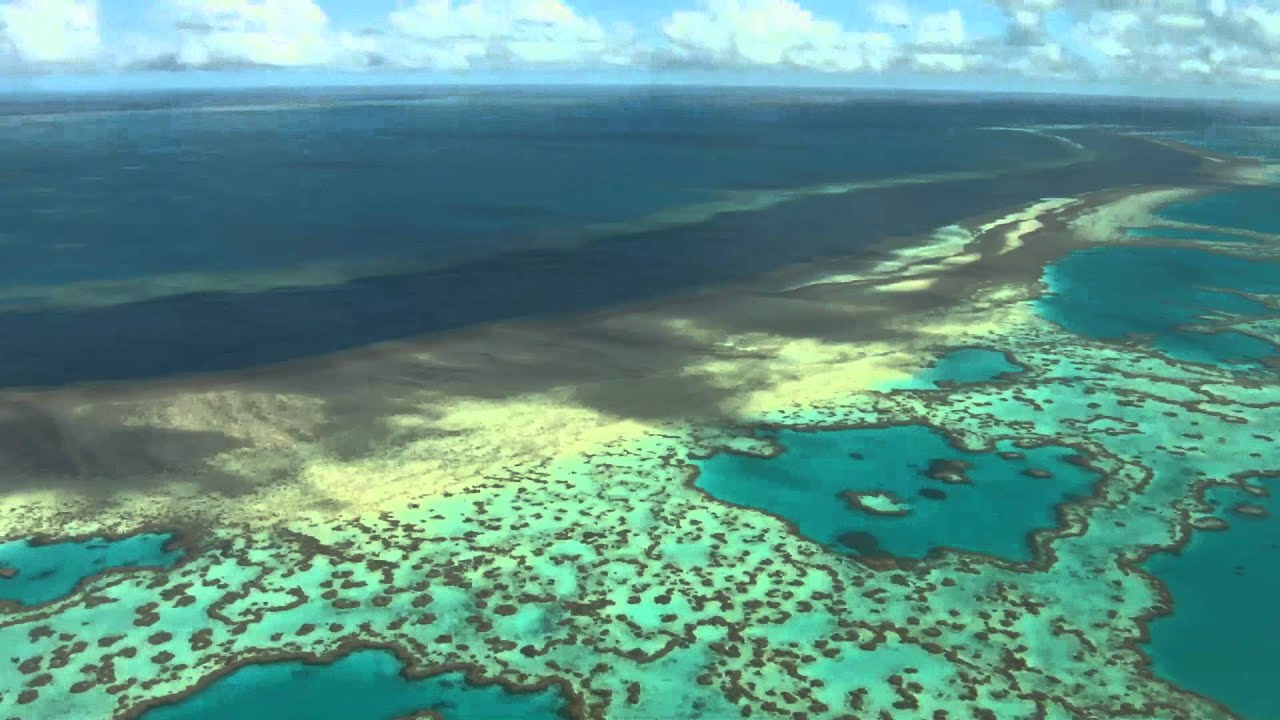This overhead aerial photograph captures an expansive and serene coastline, reminiscent of a breathtaking painting. The deep blue ocean seamlessly transitions into a lighter shade of blue as it nears the shore, where the water meets a broad stretch of dark brown sand, interspersed with patches of white sand forming wavy, chaotic patterns. Fluffy white clouds dot the clear, light blue sky, enhancing the tranquility of the scene. Seafoam, turned from white to light blue upon reaching the sand, creates fascinating patterns dotted with mysterious spots, possibly shells. Beyond the sand, shallow water exhibits a vibrant palette of bright blue and teal-green, peppered with brown spots that suggest coral. In this peaceful, untouched landscape devoid of buildings, vehicles, or people, a single wave curves gracefully along the shoreline, adding to the serene beauty of the scene.